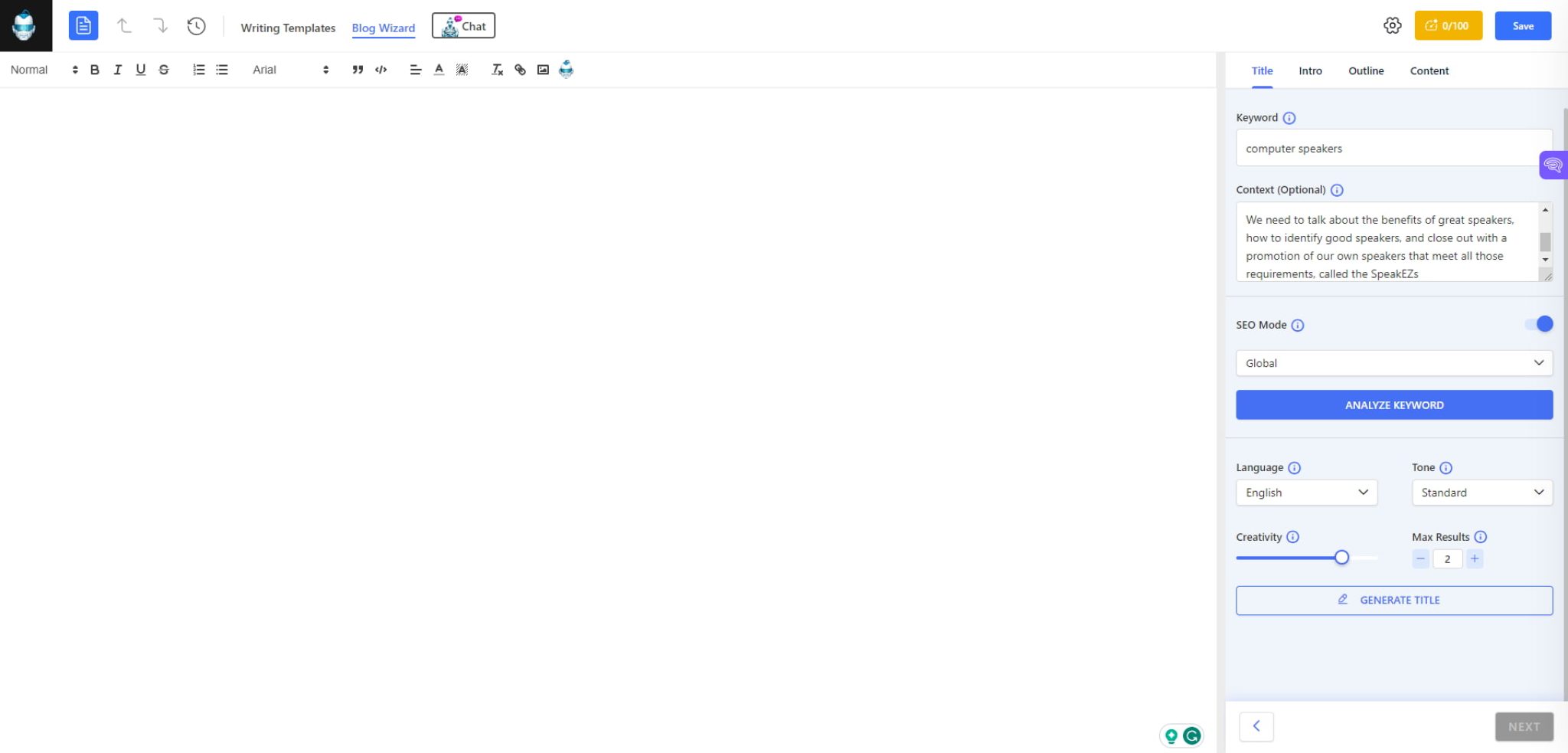The image shows an AI writing assistant interface with various editable settings and input fields. At the top, a partially obscured logo remains indistinguishable. Below it, a black section with a grayish center features another blue, unclear logo, accompanied by an up-and-down arrow for navigation or toggling settings.

Highlighted in the main view is a "Writing Template" section under the "Being Wizard" category, with a "Chat" option listed below it. The font settings are visible, configured to Arial in normal style, though the font size isn't specified.

On the right side of the interface, there are separate tabs labeled "Title," "Intro," "Outline," and "Content," suggesting that users can fill these sections to generate content, possibly with AI assistance. The interface also includes a "Keywords" section displaying "computer speakers," an optional content input field, and additional settings like LED mode.

Users are given options to save their progress or discard it using the "Save" and "Trash" buttons, respectively, based on their satisfaction with the produced content.